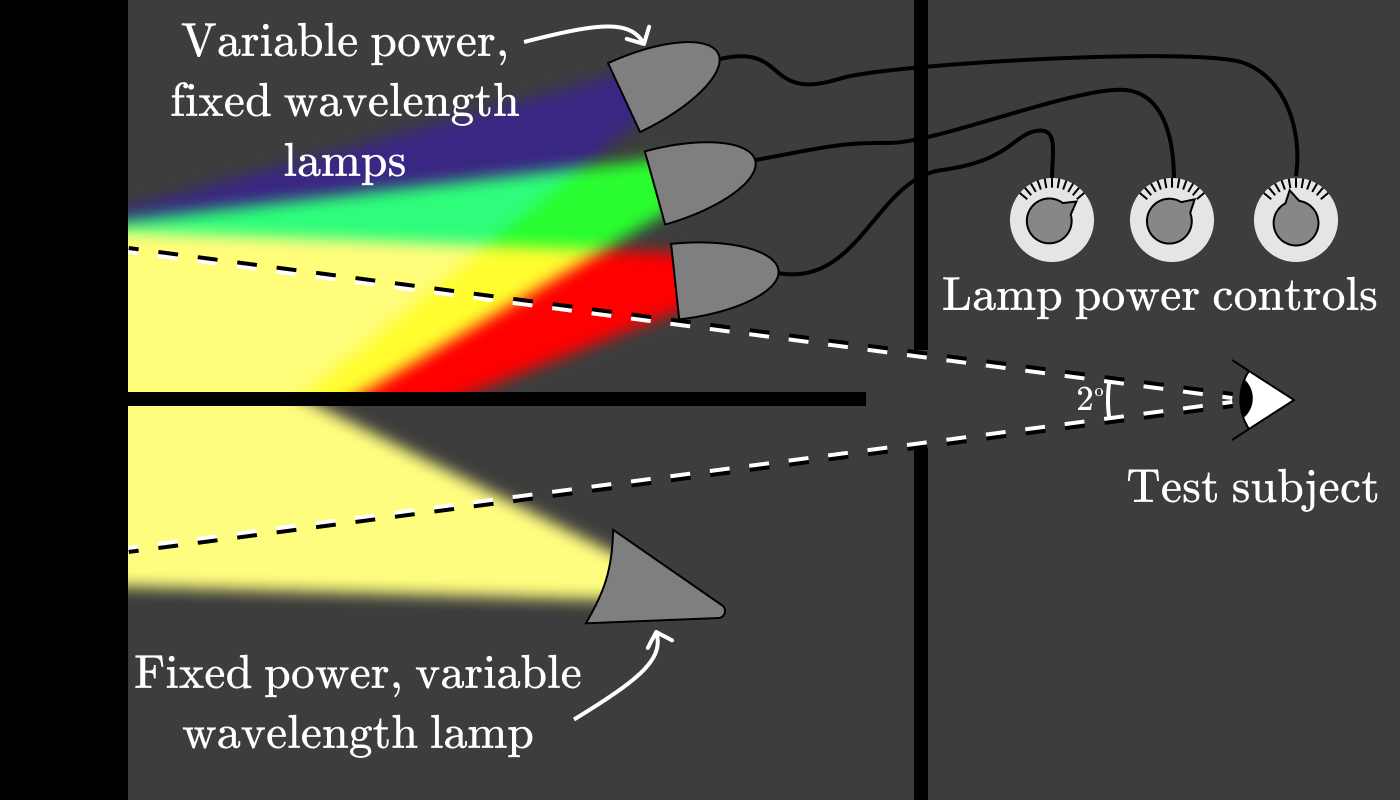The diagram illustrates a lighting setup and control mechanism, highlighting both fixed and variable properties of lamp power and wavelength. On the far left-hand side of the image, a black bar denotes the boundary of two separated rooms. In the upper portion of the image, three dome-shaped lamps labeled as "Variable Power Fixed Wavelength Lamps" emit different colored lights: blue, green, and red. These colored lights intersect to form yellow light. Below these, a single cone-shaped lamp labeled "Fixed Power Variable Wavelength Lamp" emits yellow light. The lamps are controlled through three dials labeled "Lamp Power Controls," situated above a section marked "Test Subject." Dotted lines creating a V-shape converge towards the "Test Subject" area, emphasizing the focus of the light setup on the subject. The entire diagram has a gray background, enhancing the visibility of the various elements and their connections.